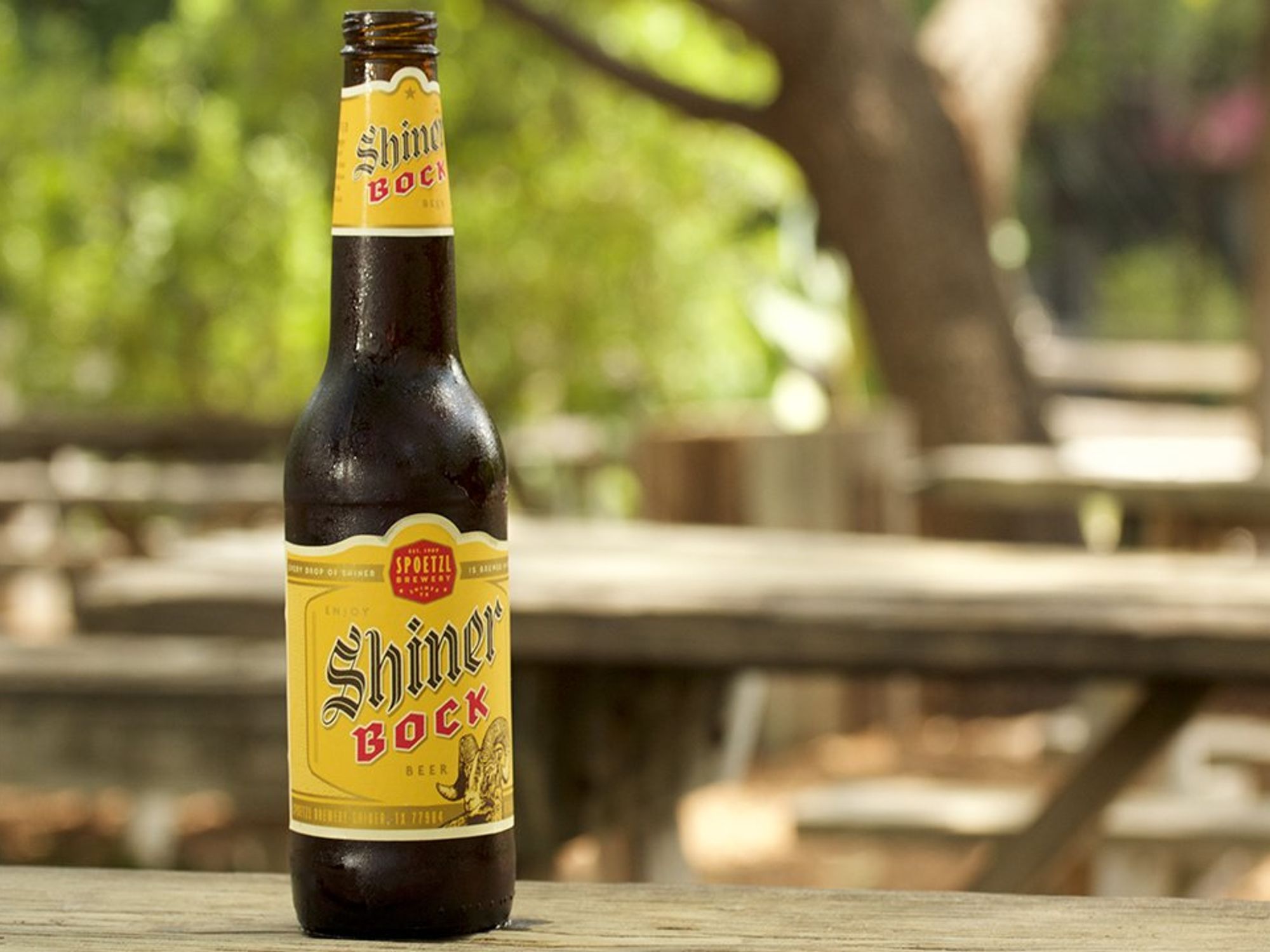In this image, the focal point is a dark-colored, imported beer bottle prominently placed on the left side of the frame. Adorned with a distinctive yellow label, the bottle displays the text "Shinner Rock Beer" and features an illustration of an animal that appears to be either a ram or a goat. The beer bottle, covered with condensation, suggests that it is very cold. The setting appears to be a park, with park benches and tables faintly visible in the background. The surrounding environment includes various green bushes and a tree on the right side, although the background remains quite blurry, emphasizing the beer bottle in the foreground. The bottle rests on a gray table, adding a contrast to the overall scene.